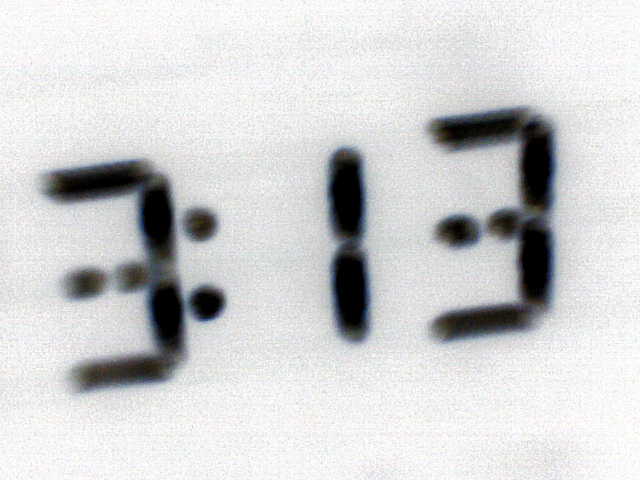The image depicts a digital clock or watch against a stark white background. The display shows the time as "3:13." The time is rendered in a classic digital font, characterized by its block-like rectangular shapes. The number "3" is constructed with a single horizontal line at the top, two vertical lines descending from either end, and another horizontal line at the bottom, creating a slight separation in the middle. The colon separating the hours and minutes consists of two vertically aligned dots. The number "1" features two short horizontal lines stacked vertically. The digits are black, providing a sharp contrast against the white backdrop.